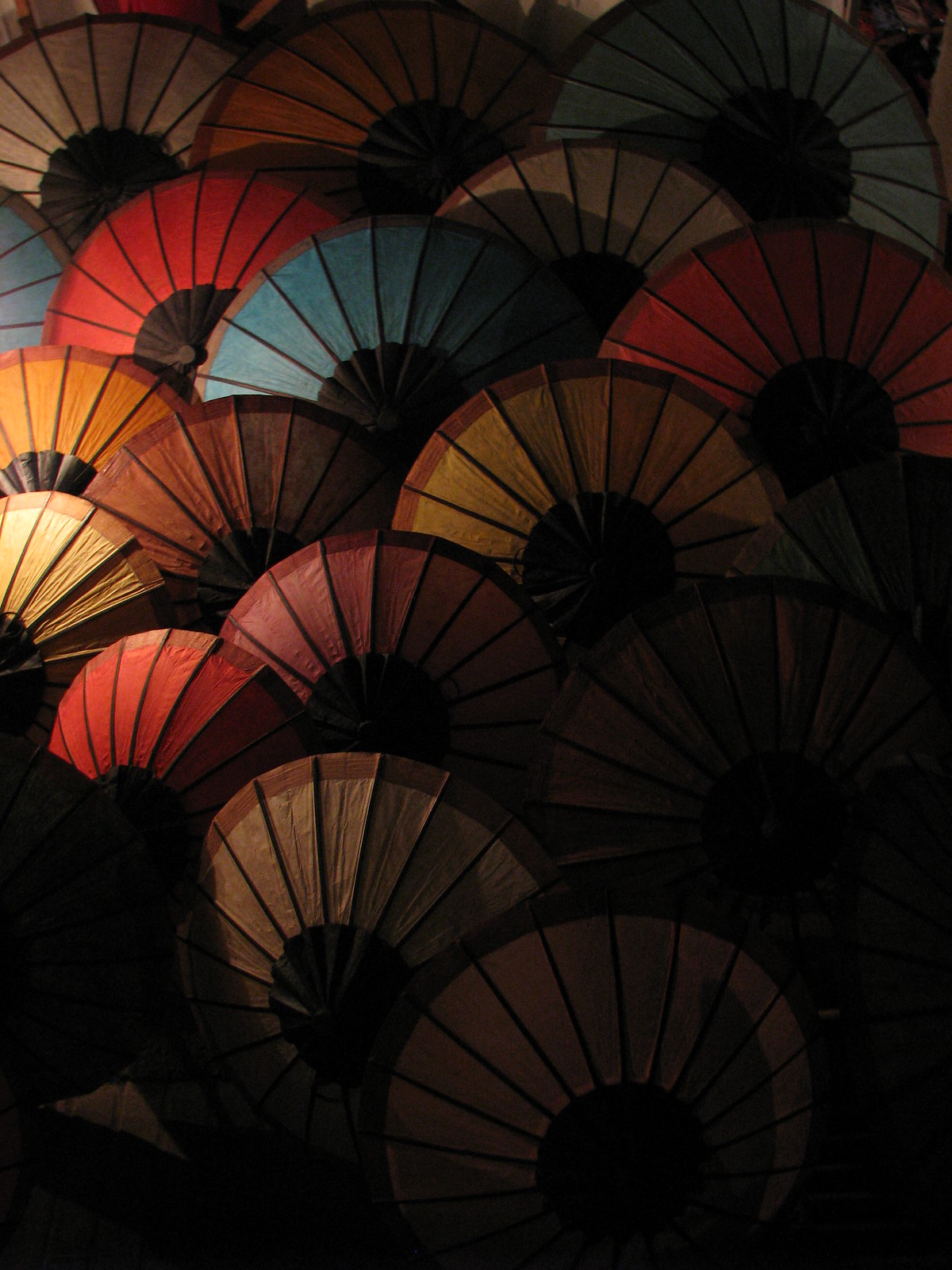This photograph captures an overhead view of a multitude of open umbrellas, creating a captivating and colorful tapestry. The umbrellas, showcased with their tops facing the viewer, come in a variety of hues including beige, pink, red, brown, tan, yellow, hot pink, baby blue, cyan blue, orange, and mixtures of lighter blue and white. Each umbrella is detailed with a small black circle near the edge, resembling a central riveting point, though handles are not visible. The lighting in the image is starkly divided; the bottom section is very dark and shrouded in shadow, while the top center is brightened by a light source on the left, creating a dramatic cascade of light and shadow over the array. The overlapping umbrellas, set against a partly visible tile floor, appear strategically arranged as if part of a choreographed routine, suggesting the presence of people beneath them. This intricate interplay of colors, lighting, and composition makes for a visually striking and detailed scene.